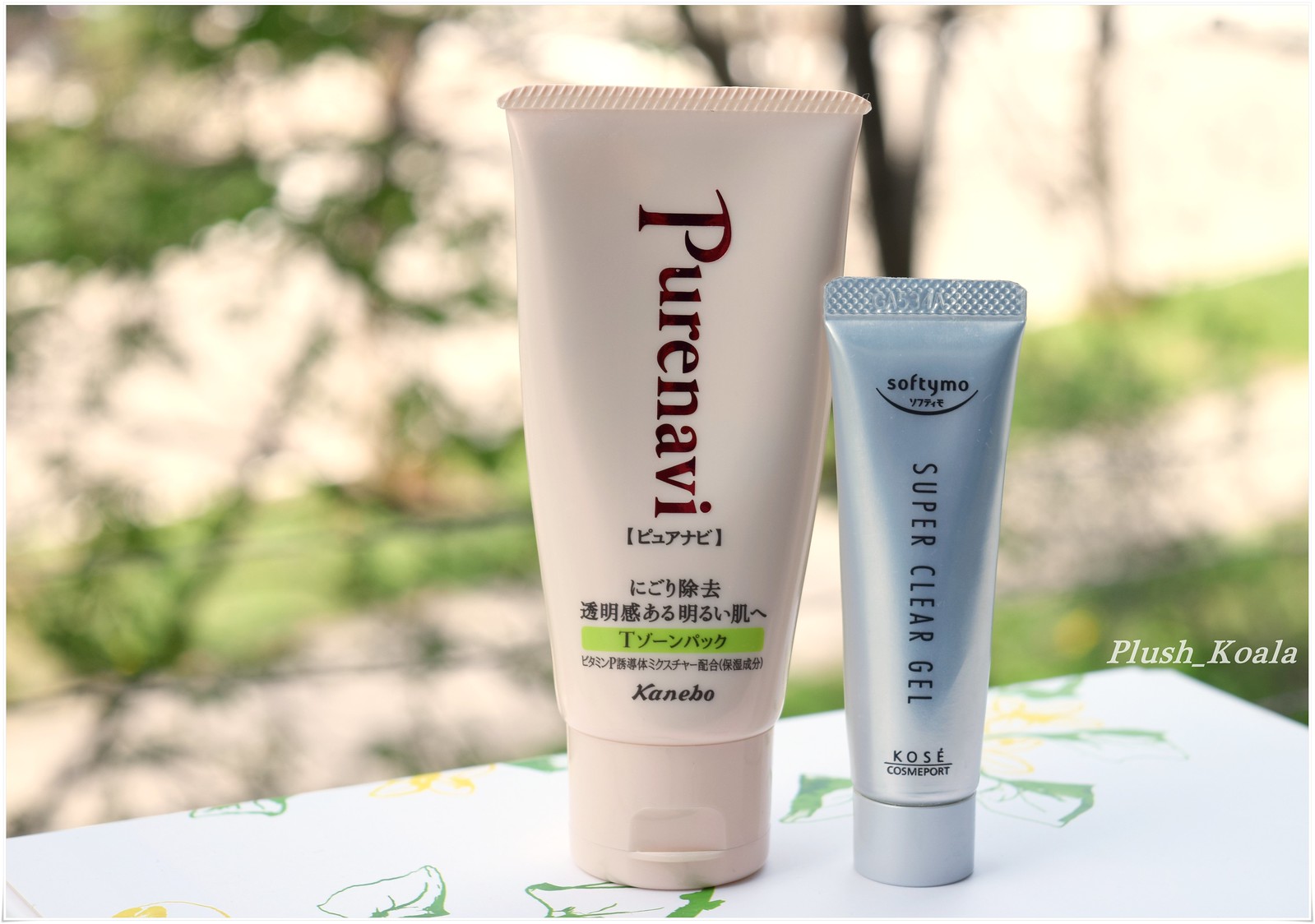The image depicts two cosmetic products standing upright on an outdoor table with a floral design. The background features vibrant greenery, including trees illuminated by sunlight. The product on the left is a white tube labeled "Purnavi," with additional text in Chinese characters. Near the base, it also features the brand name "Kanibo" within a green bar accompanied by more Chinese writing. The smaller product on the right is a blue tube branded "Soft YMO," and labeled "Super Clear Gel." At the very bottom, "Cosay Cosmoport" is printed. Both tubes are capped and placed securely, suggesting a serene and natural setting for showcasing these beauty products.